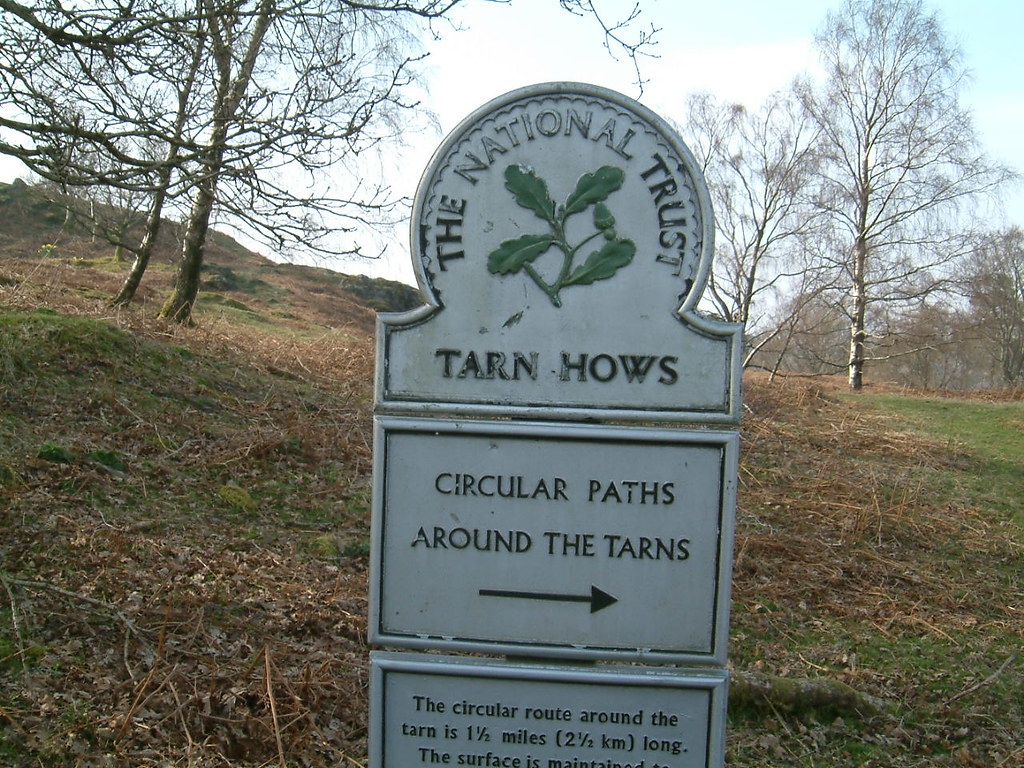The image features a tall, curved metal marker approximately four to five feet in height, prominently displayed on a grassy hill surrounded by barren trees. The marker itself is white with red print and divided into three sections. The top panel, with a rounded top, reads "The National Trust" and features a painted depiction of leaves on a branch. Just below, the second section reads "Tarn House" followed by "Circular paths around the tarns" with an arrow pointing to the right. The final visible part on the lower panel indicates, "The circular route around the tarn is one and a half miles, two and a half kilometers long. The surface is…" before being cut off by the photo's border. The setting appears to be in late autumn or early spring due to the brown foliage on the ground and the leafless trees. The hill slopes downward to the right, and the scene is framed by a mix of shrubs, grass, and weeds, highlighting a serene yet slightly desolate landscape.